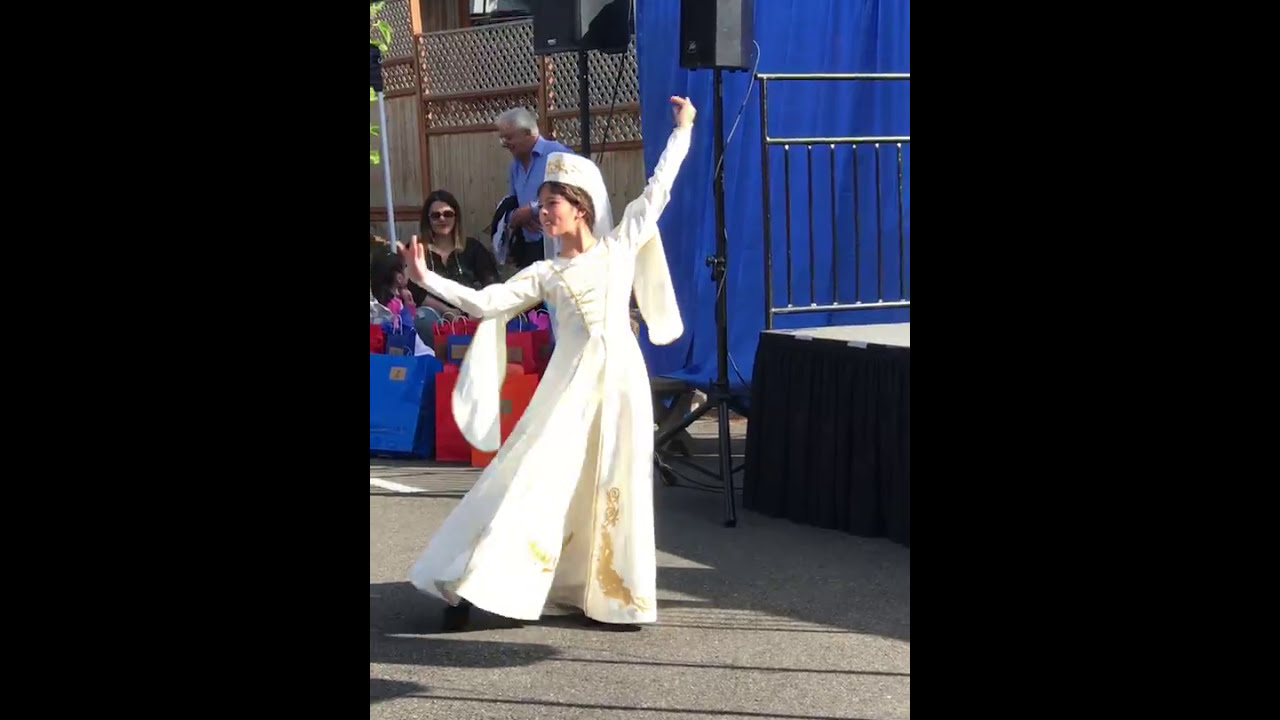The image captures an outdoor scene featuring a performer dressed in an elaborate, white and gold costume with long sleeves and a full, flowing bottom. She has one arm raised and one arm lowered, complementing her poised stance. Her head is adorned with a distinctive white hat. Her light-colored hair cascades under the headpiece. The setting includes a textured gray pavement area where she performs. Behind her, a stage stands with a blue curtain and black skirting, accompanied by speakers and brown fencing. In the background, a man with gray hair in a blue button-down shirt is standing, while a woman with glasses sits nearby, looking towards the dancer. The scene also includes various bags, possibly gift bags, adding to the overall festive atmosphere.